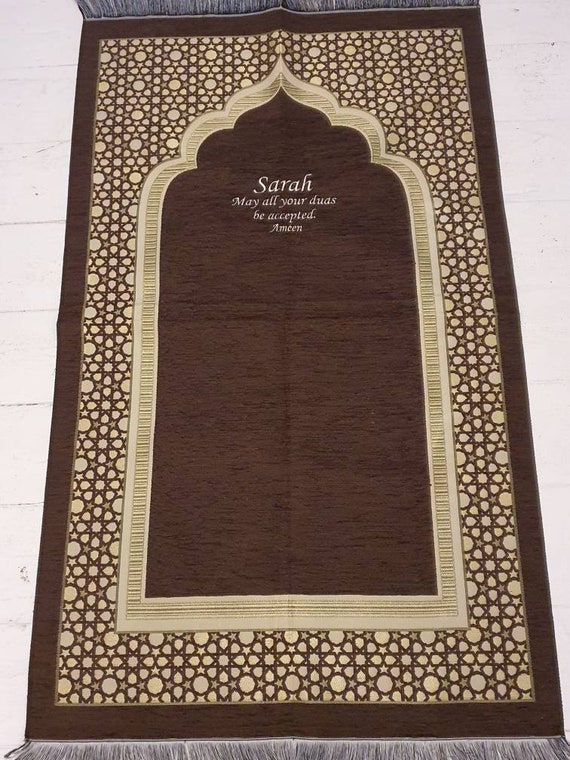The photograph displays a detailed color image of a vertical, rectangular prayer rug positioned on a white tile surface. The rug features a dark brown border with white fringes along the top and bottom edges. Enclosed within the border is a geometric, leaded glass pattern made up of rows of large tan circles interspersed with smaller circles and black lines, creating a stars-and-circles motif. There are eighteen rows and ten vertical columns of these circles.

At the center of the rug is a prominent dark brown rectangle that resembles a window with a Moroccan arch at the top, outlined in wide, textured gold trim. Inside this dark brown rectangle, near the top, the name "Sarah" is written in large, elegant white script. Below this, in smaller white text, it reads, "May all your duas be accepted. Amin." The intricate patterns and symbolic elements suggest the rug's potential use in Islamic prayer or as a decorative piece inspired by Islamic art.